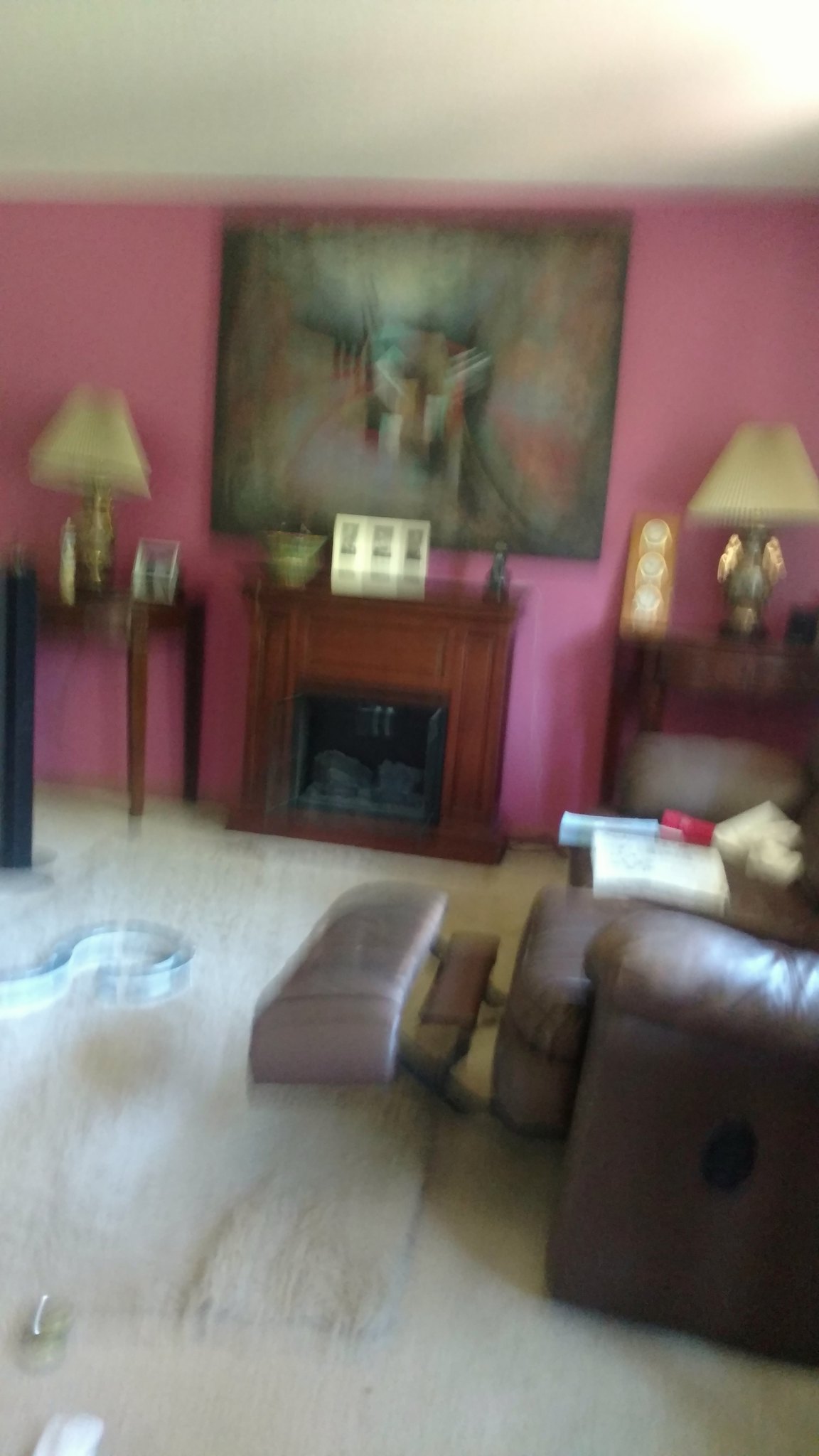The photograph is a vertical, first-person perspective snapshot of a blurry living room, likely taken with a handheld phone camera. At the top, a white ceiling with shadows gives way to a vivid Pepto-Bismol pink wall. This wall features a large, indistinguishable piece of art above a small electric fireplace, which is flanked by wooden sides. The fireplace mantle holds several unclear items, possibly framed photos, knick-knacks, and a bowl or planter. To the left of the fireplace is a wooden side table, nearly as tall as the mantle, holding a lamp and other fuzzy objects. To the right, another table with a different lamp and more indistinct items can be seen. The floor is very light-colored, possibly white carpet, with an area rug adding texture. A brown leather reclining chair with an extended footrest and potentially some papers or a book on its right arm is visible on the right side of the image. The entire scene is extremely blurry, suggesting motion when the photograph was taken.